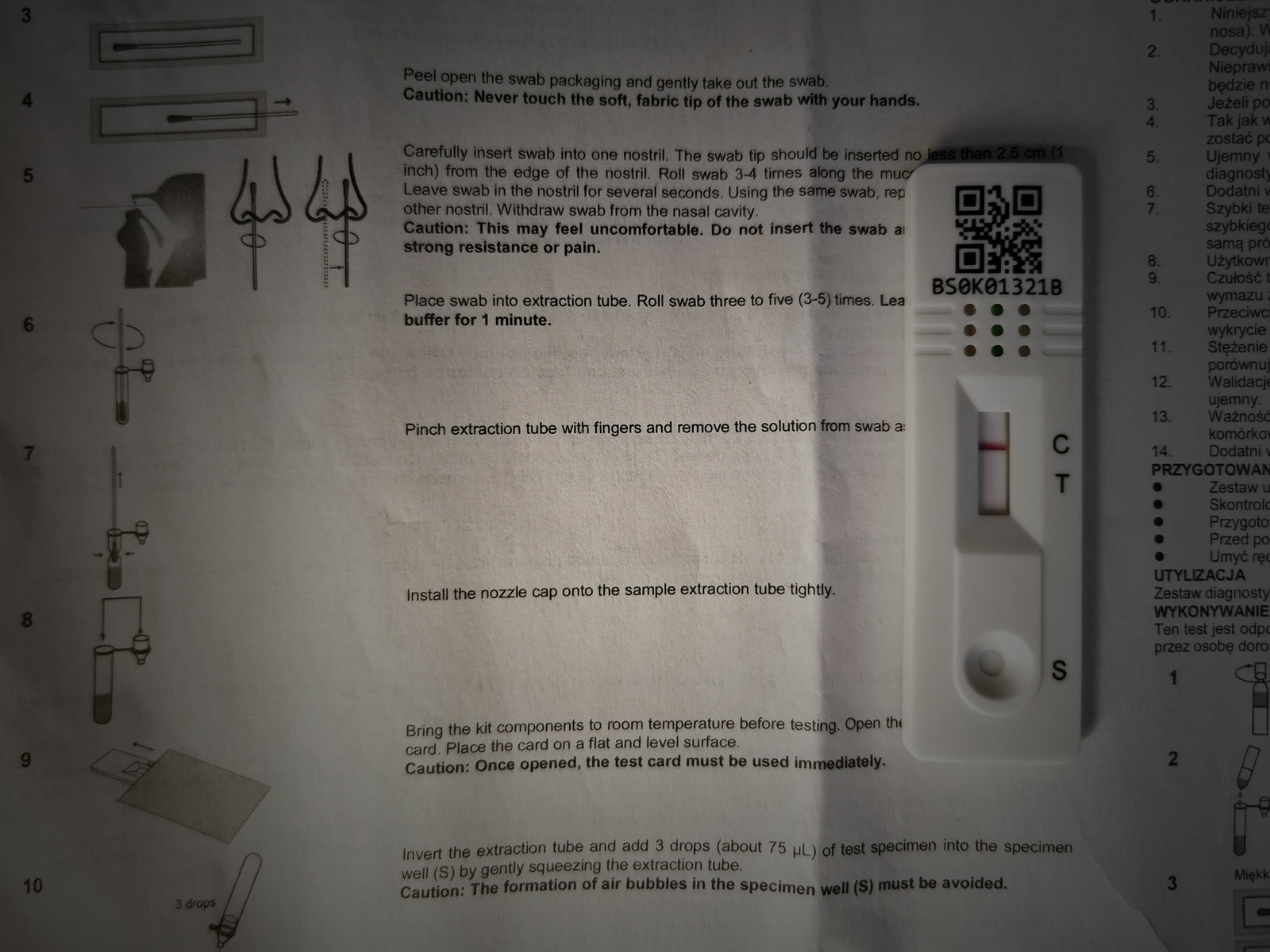The photograph depicts a COVID-19 test kit placed on top of its printed instructions. The image is somewhat dark, emphasizing the contrast between the white test kit and the surrounding text. To the left side of the picture, instructional icons illustrate the proper technique for inserting and swirling nasal swabs in the nasal passages.

The accompanying detailed text instructs: "Carefully insert the swab into one nostril. The swab tip should be inserted approximately one inch from the edge of the nostril. Roll the swab three to four times along the inner nasal walls. Leave the swab in the nostril for several seconds. Using the same swab, repeat the process in the other nostril. Withdraw the swab from the nasal cavity. Caution: This may feel uncomfortable. Do not insert the swab if you encounter strong resistance or pain."

To the right of these instructions lies the actual test kit, a white plastic rectangular device. It features a barcode at the top, labeled BS0K01321B. In the middle of the rectangle, there is an indicator window with markings 'C' and 'T' next to it. A red arrow points to the 'C' mark, indicating the control line. At the bottom of the device, a small round indentation is labeled with an 'S', which stands for the sample application spot.